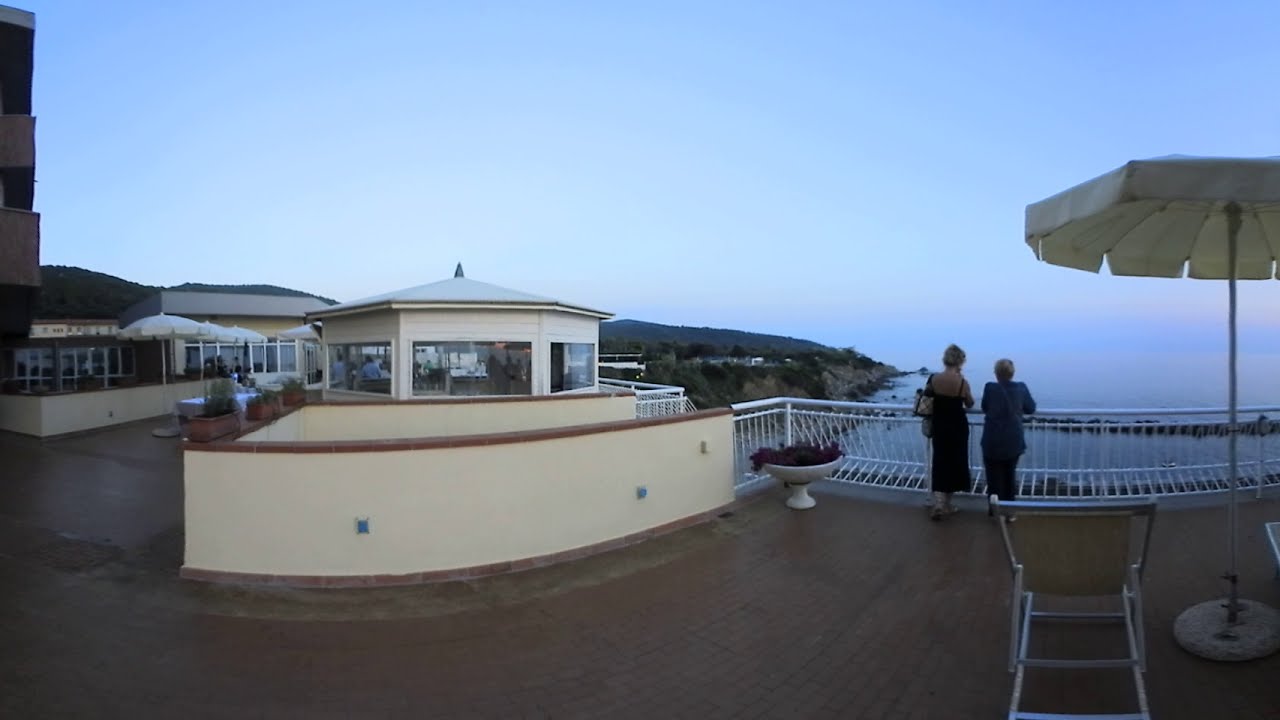The image showcases a fisheye view of an outdoor setting on a raised balcony overlooking the ocean. Central to the scene are two people, possibly women, standing by a white metal railing, gazing out at the vast water expanse and blue horizon. To their right is a sun umbrella positioned horizontally on a stand, shading a chair beneath it. The ground beneath them is a rust-colored brick surface, enhancing the cozy atmosphere.

To their left, a white flower pot filled with vibrant pink flowers rests on the ground. Beyond the pot stands a distinctive octagonal building with glass windows and wood accents, resembling a gazebo or part of a restaurant. Additional umbrellas and stands can be seen in front of another structure further along the balcony. To the far left, three brownish boxes and some windows are visible, contributing to the overall picturesque setting. The backdrop features undulating hills that lead into the serene ocean, completing this scenic coastal view.